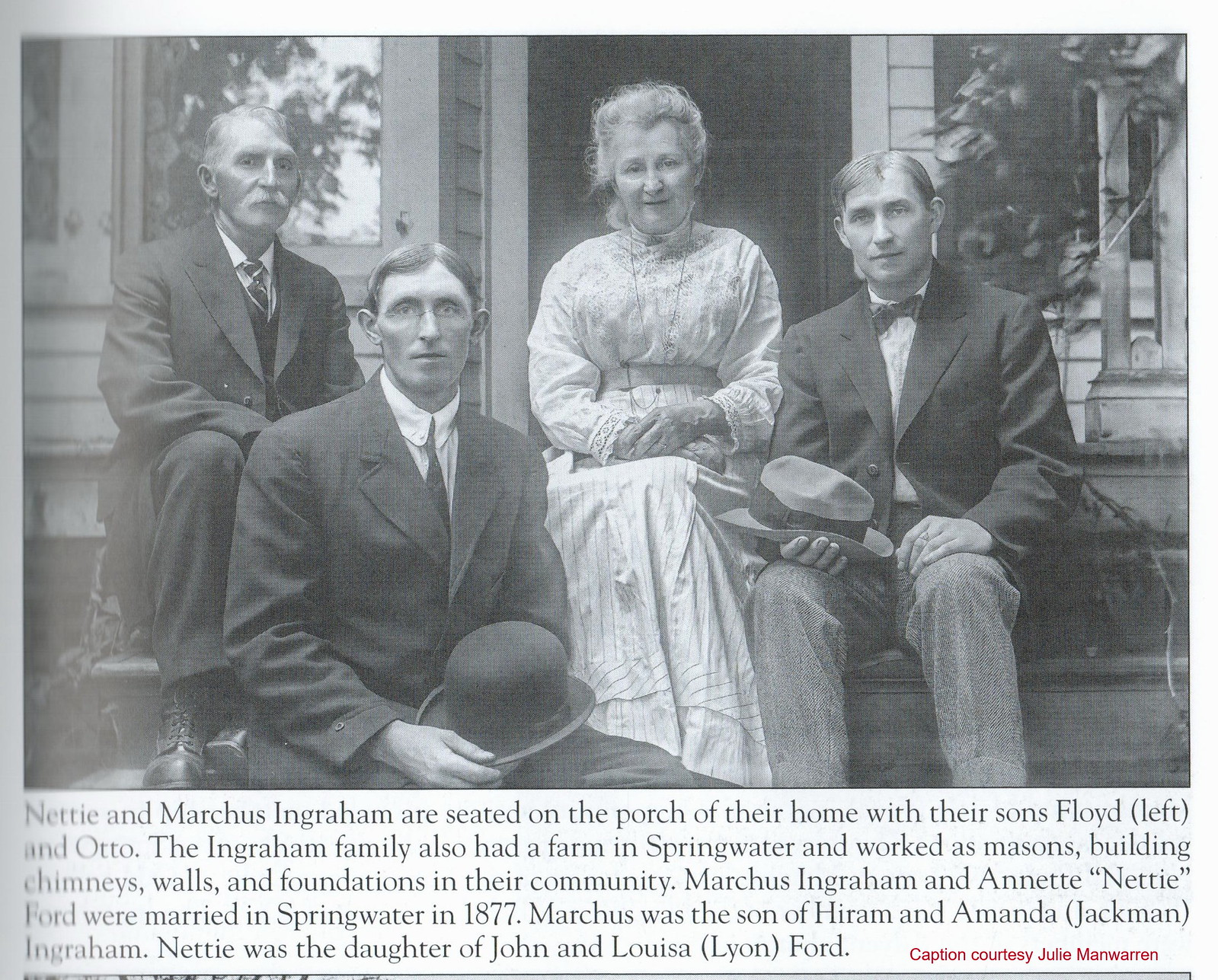This is an old black-and-white newspaper clipping featuring a vintage photograph from the 1800s, depicting four people seated on the steps of a house, identified as Nettie and Marcus Ingram with their sons Floyd and Otto. On the top left is an older gentleman with a white mustache, wearing a suit, identified as Marcus Ingram. Sitting in front of him is another man, slightly younger, wearing glasses and holding a top hat, likely one of their sons. To their left sits an older woman in her 70s, dressed in a white dress with her arms folded in her lap, identified as Nettie Ingram. To her left, another middle-aged man, dressed in a suit and bow tie and holding his hat, represents the other son. The bottom of the image states that Nettie and Marcus Ingram were married in 1877, and Marcus was the son of Hiram and Amanda Jackman Ingraham, while Nettie was the daughter of John and Louisa Leon Ford. The Ingram family owned a farm in Springwater and contributed to their community as masons. The bottom right corner of the photo contains the caption "courtesy of Julie Mann Warren."